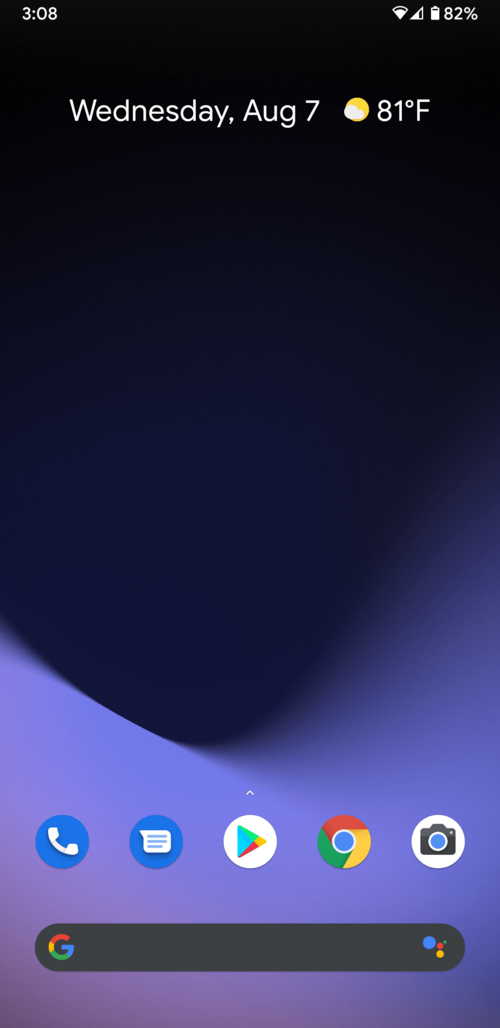The image is a screenshot of a home screen in portrait orientation on a smartphone. In the upper left corner, it displays the time as 3:08, and in the upper right corner, the battery level is shown to be at 82%. Below this, the date and weather information are displayed, reading "Wednesday, August 7th" accompanied by a partly cloudy icon and a temperature of 81 degrees Fahrenheit.

The background features a gradient that transitions from almost black at the top, through dark navy blue, to lighter shades of blue, curving into pink and violet hues as it moves down towards the bottom. The colors blend together in an abstract pattern, becoming progressively lighter. 

At the bottom of the screen, there are five icons arranged horizontally: Phone, Messaging, Google Drive, Google Chrome, and Camera. Just below these icons, a large Google search bar spans the width of the screen, ending with the colorful circular icon of Google Assistant (a small red circle within a yellow circle).

In essence, this image captures the unlocked home screen of a smartphone, presenting the user with various quick-access options such as making calls, checking messages, using apps, browsing the internet, taking photos, or interacting with Google Assistant.